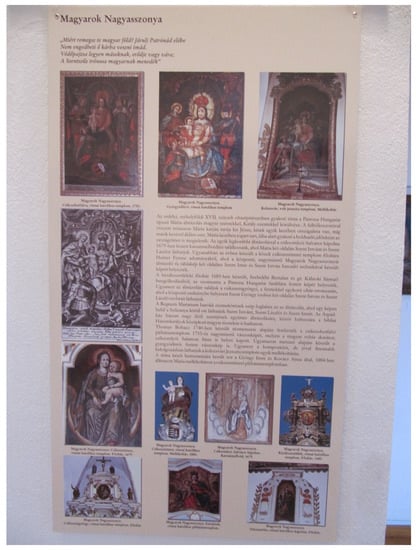The image appears to be an infographic or a page from a publication displayed on a cream background, titled "MAGYAROK NAGYASSZONYA" in bold black letters at the top. The layout features a collection of paintings and possibly photographs or stained-glass artworks, primarily depicting religious themes, particularly images of Jesus and Mary, mother of Jesus. The artworks are organized into several rows: three at the top, followed by a black and white piece on the left, four more across the next row, and three additional artworks at the bottom row. Interspersed among the images are smaller sculptures and depictions of thrones and buildings. Accompanying the images are captions that are too small to discern, as well as a few blurry paragraphs in the middle that are difficult to read. The overall presentation suggests an informative display, likely detailing the historical and cultural background of the depicted religious and ancient scenes.